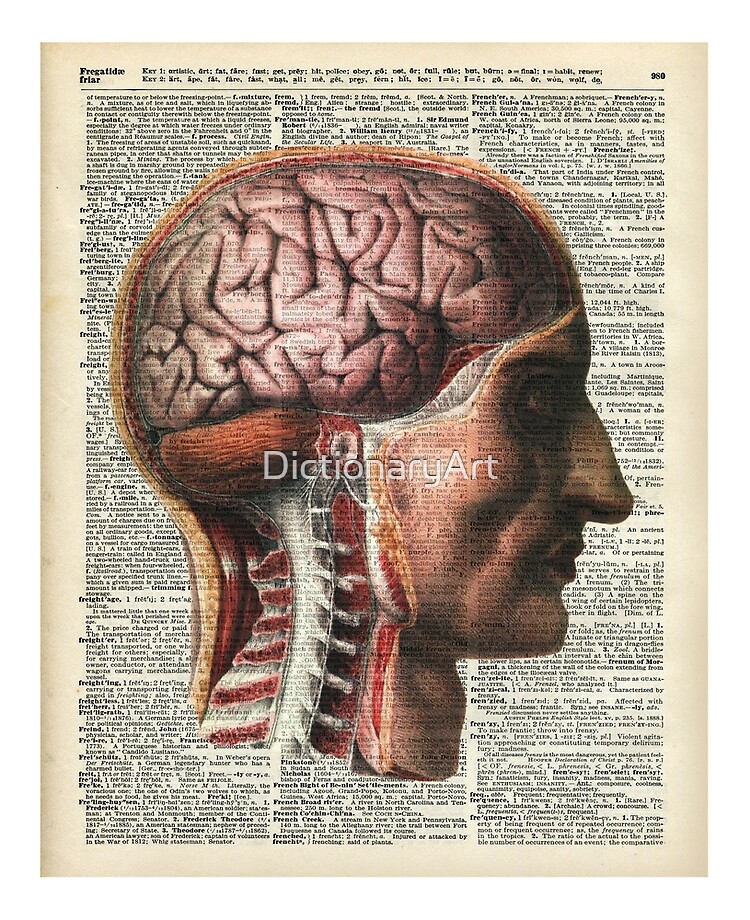This detailed scientific image features a side profile of a Caucasian man's head, showcasing both his skin and underlying anatomical structures. Displayed on an old dictionary page numbered 980, which spans words starting from "fregatidae" to "frequency," the artwork prominently illustrates his brain and spinal cord, right down to the neck vertebrae. His facial features are strong and distinct, characterized by a Roman nose, deep-set eyes, angular jaw, and pursed lips. The skin gives way to a vivid depiction of the brain and vertebrae, revealing a color palette of pink, light brown, and touches of black. Various vertebrae images surround the spine, contributing to the anatomical theme. Written across the front of the picture are the words "dictionary art," tying together this unique fusion of scientific illustration and literary background.